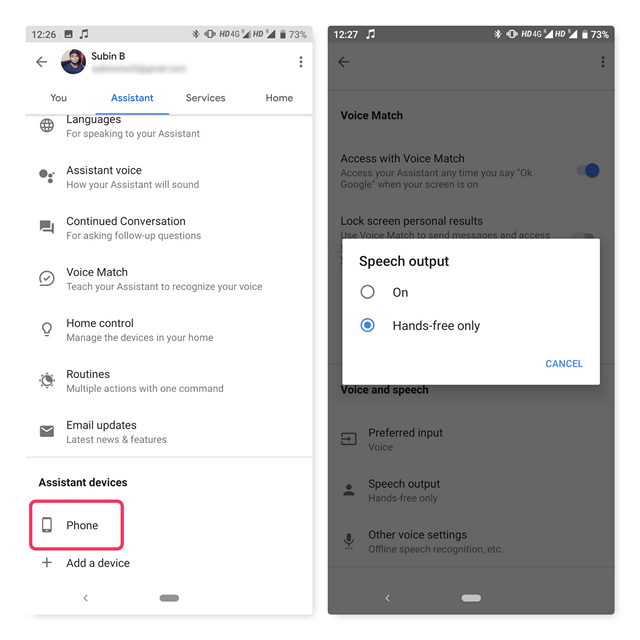Here is a detailed and descriptive caption for the provided image:

---

The image showcases two cell phone screenshots displayed side by side. 

The screenshot on the left depicts the settings menu of a smartphone's Google Assistant. 
- The current time is shown as 12:26 PM, and the battery level is displayed at 73%.
- At the top of the screen, the profile associated is labeled "Subin B" and features a profile picture where the individual is facing the camera.
- Below the profile, the screen displays a menu titled "Assistant services" with the "Home Assistant" option selected.
- A vertical list of menu items follows, including:
  - Languages
  - System Voice
  - Continued Conversation
  - Voice Match
  - Home Control
  - Routines
  - Email Updates
- Below these options, a section titled "Assistant devices" is shown, with the "Phone" option highlighted with a red frame.

The screenshot on the right displays a pop-up window titled "Speech Output."
- The pop-up contains two radio buttons for different options:
  - "On"
  - "Hands-free only"
- The "Hands-free only" option is selected.

---